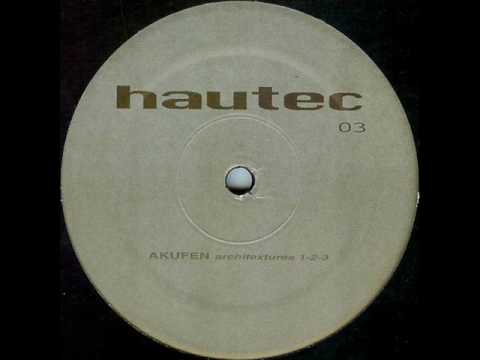The image is an up-close shot of a vinyl record label, presented in a rectangular frame. Dominating the center is a large, aged cream-colored circle that extends to touch both the top and bottom centers of the image. In the middle of the circle is a small hole, designed for placement on a record player spindle. The top of the circle features the word "HAUTEC" in prominent brown font, and situated just below the ‘C’ is the number "03". Directly below the center hole, the text "AKUFEN" appears in all caps. Surrounding the circle, the remainder of the image is filled with the deep black of the record. Additional faint text under "AKUFEN" seems illegible, followed by the sequence "1-2-3" in small writing.